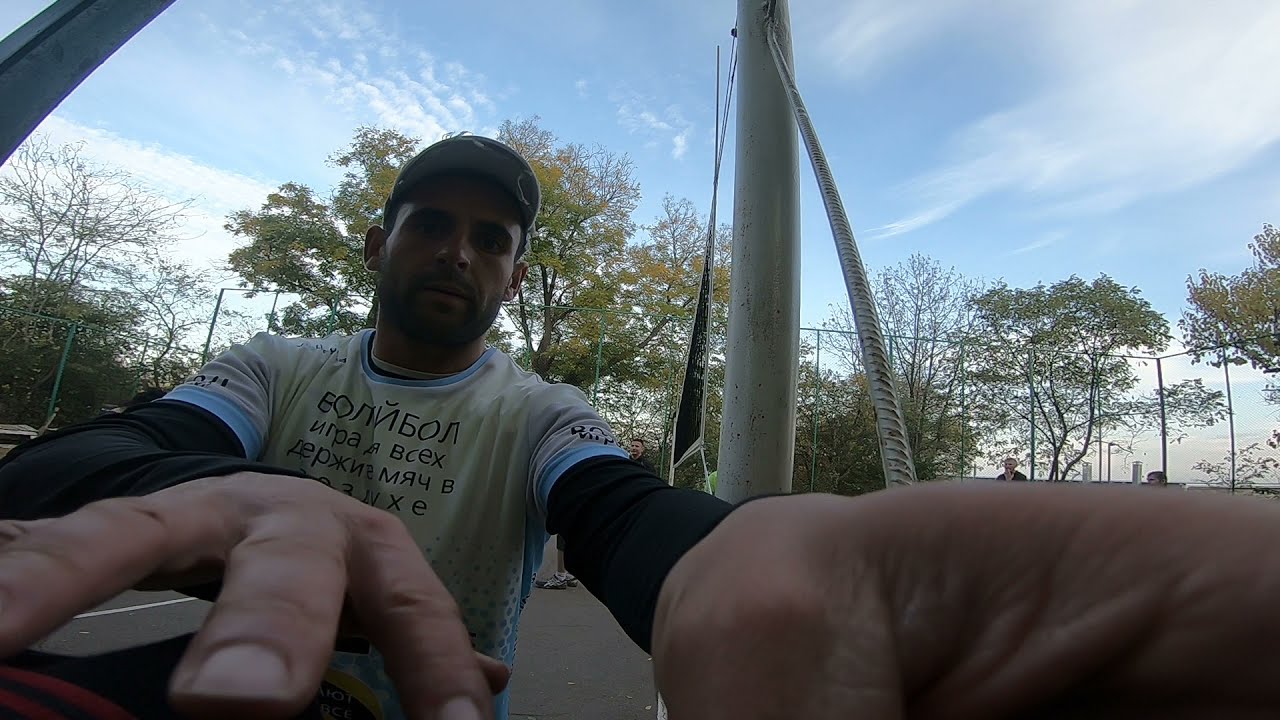The photo depicts a man outdoors on a sunny day with a slight overcast sky, characterized by pale blue hues and feathery white clouds. The man, who appears to be trying to take a selfie or adjust the camera, faces the viewer with a serious expression and has a light beard and mustache. He dons a baseball cap and wears a distinctive pale yellow and pale blue T-shirt adorned with black symbols and text in a non-English script, layered over a long-sleeved black undershirt. His hands are distorted and stretched out toward the camera, with his right hand positioned in the lower left and his left hand in the lower right of the image. The background features a tall pole, possibly a flagpole or a volleyball net pole, and a tall fence with trees rising behind it, creating a layered backdrop against the broad stretch of sky. The scene appears to be set on an asphalt surface, enhancing the outdoor atmosphere.